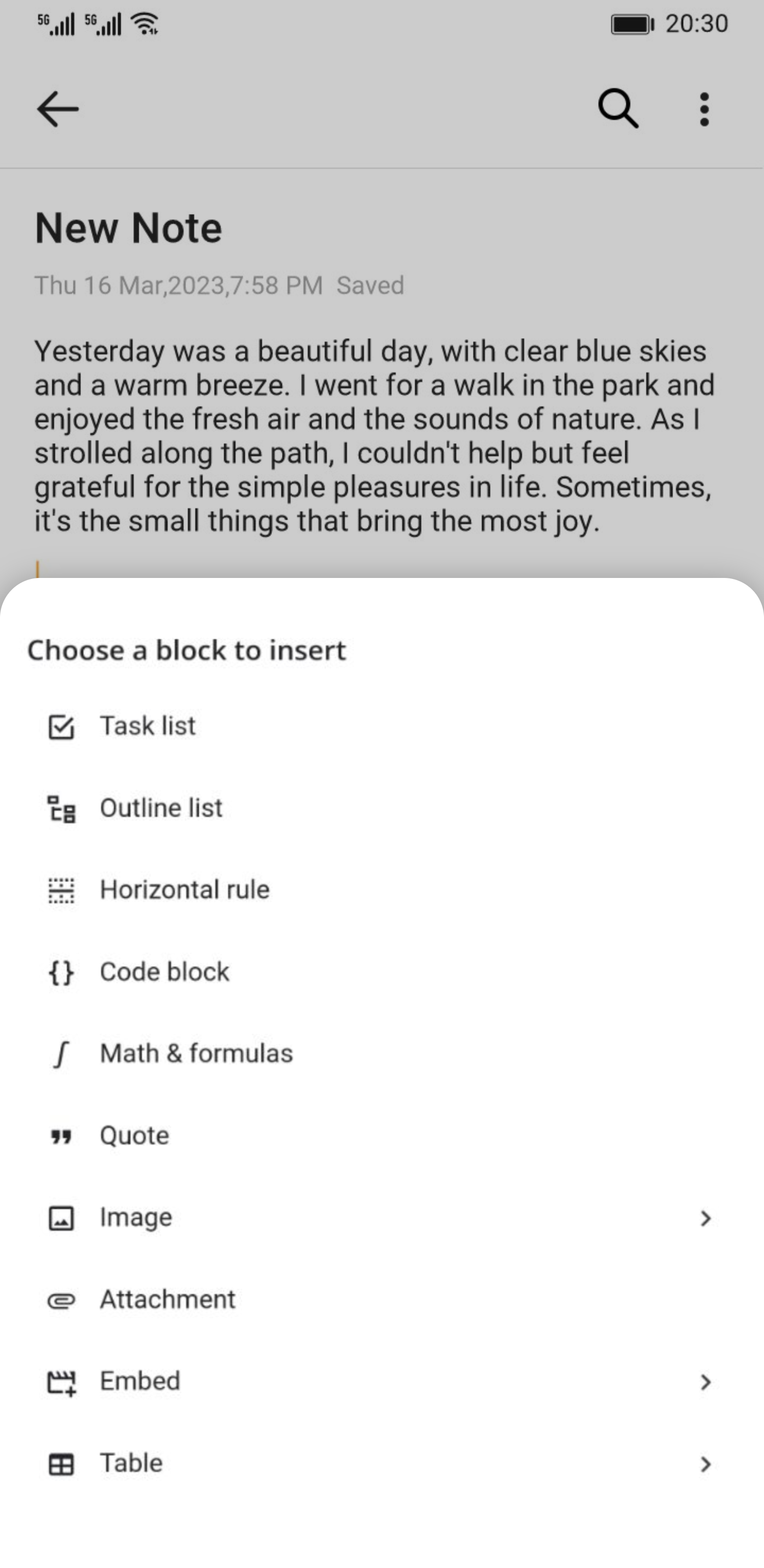This screenshot captures a note-taking application interface with an opened menu overlay. At the top of the screen, a back button is positioned on the left, while a search button and a "More Info" option, represented by three vertical dots, are aligned on the right. Just beneath this header, the text "New Note" appears on the left side, indicating the title of the current note. Below the title, the note content area is visible. 

A white menu, which has been pulled up from the bottom, dominates the lower portion of the screen. This menu is titled "Choose a Block to Insert" and offers multiple block options indicated by icons on the left and text labels on the right. The available options include: Task List, Outline List, Horizontal Rule, Code Block, Math and Formulas, Quote, Image, Attachment, Embed, and Table. The menu features dark gray text on a white background, ensuring clarity and readability.